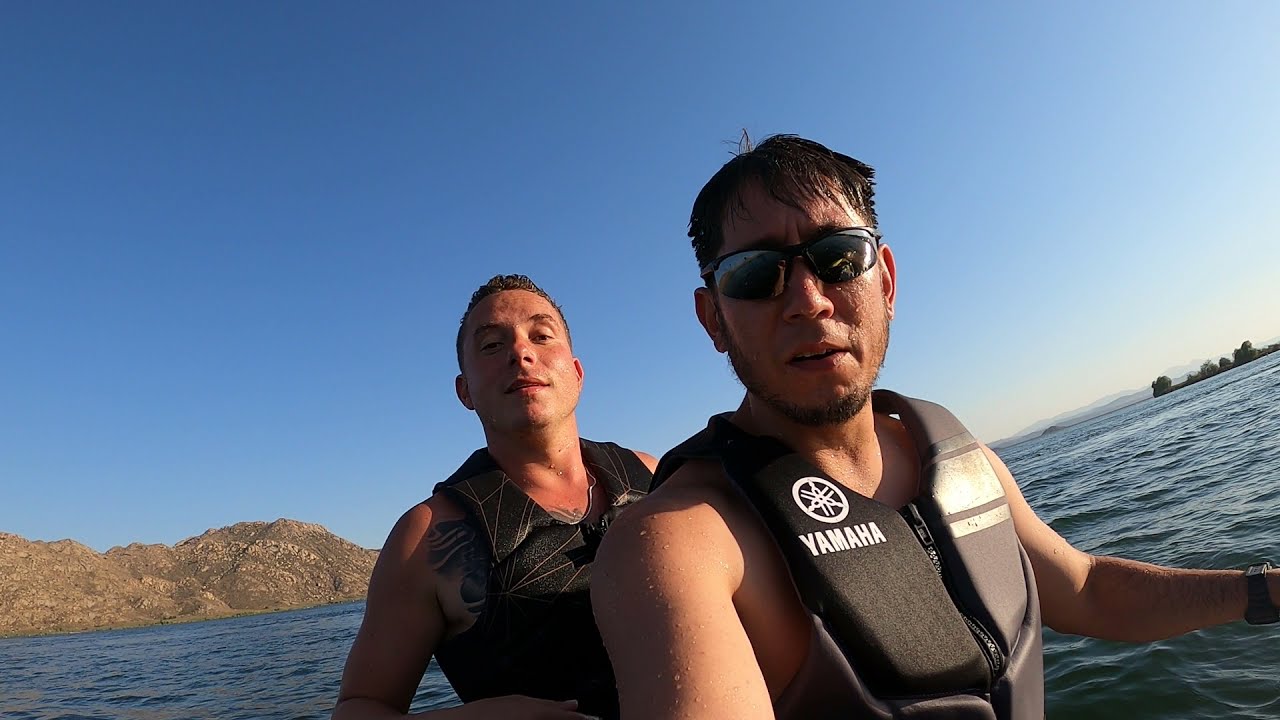The horizontally aligned rectangular image captures two men on a deep blue body of water, possibly in a canoe or kayak. Both men, centered in the photo, are wearing life vests and appear wet, indicating recent contact with the water. The man in the front has wet, short black hair, black sunglasses, and short stubble around his beard area. He is staring at the camera with his mouth slightly open. His life vest, which is identifiable by the white Yamaha logo, reveals that he is shirtless. Behind him sits a man with short brown hair, a large tattoo on his chest, and a black vest featuring thin gray lines. This man is also looking slightly downward with his mouth open, appearing Caucasian, in contrast to the possibly Asian or Hispanic front man. The background beautifully showcases a brown, rocky cliff side, dark blue water, a clear blue sky, and distant trees on the right, suggesting land nearby. The overall setting conveys an outdoor, possibly midday adventure with clear weather and lingering natural beauty.